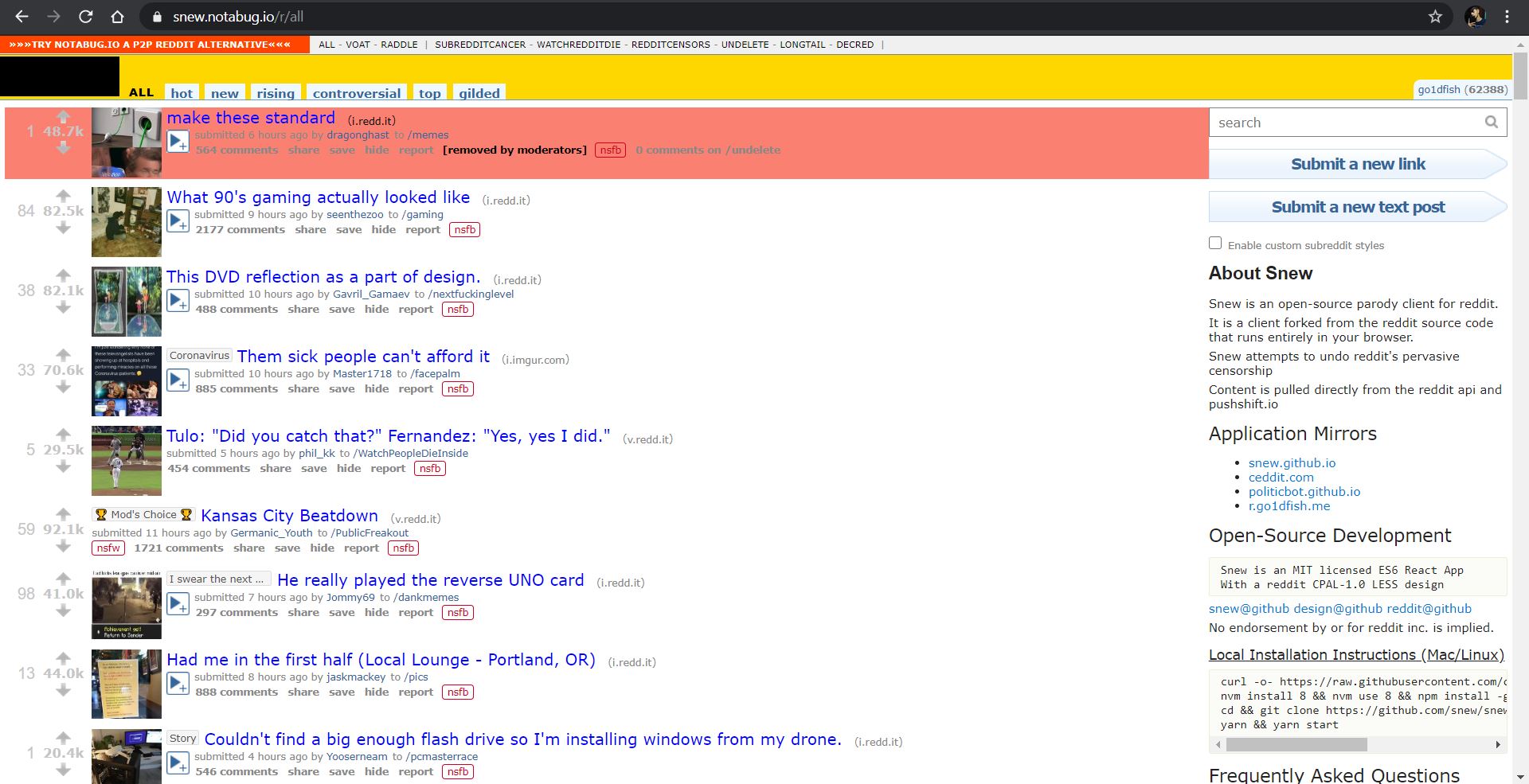The image appears to be a screenshot of a Reddit-like website. Across the top of the page, there is a black navigation bar and just below it, a yellow bar featuring navigational links labeled “all,” “hot,” “new,” “rising,” “controversial,” “top,” and “gilded.” The primary content area consists of a series of posts represented by small square thumbnails and text descriptions.

At the top of the list, there's a highlighted post in red, although its content isn't fully identifiable, it seems to say "make these standards." Next to this, there are both blue and red text elements, alongside some black text.

Down the list, other posts include titles like "what 90s gaming actually looked like" and "DVD reflections part of design," each accompanied by a small image. Additional posts display titles like "Them slick people can't afford it," which likely indicates a meme, followed by "Chulo, do you catch that? Fernandos, yes I did," appearing to be a humorous or meme-related post, possibly related to sports. Another notable post reads "Kansas City beat down," lacking any accompanying image.

Further posts feature titles such as "he replays the reverse Uno card," accompanied by another image, and "had me, the first top, local lounge Portland OR." One of the concluding posts discusses a humorous anecdote: "couldn't find a big enough flash drive, so I'm installing Windows for my drone."

To the right-hand side of the content area, there is a sidebar with more site options and information, confirming the platform is indeed Reddit. This sidebar includes options like “submit new link” and “submit a new text post,” and describes "Snu," an open-source parody client for Reddit designed to counteract Reddit's censorship. The sidebar also mentions "Snu" is a forked client that operates within a web browser, pulling content from Reddit and a service called pushshift.io. There is a segment about local installation instructions and frequently asked questions, though this part is cut off and not fully readable.

Overall, the image illustrates a dynamic feed of user-generated content typical of Reddit, emphasizing memes, user posts, and a detailed navigation and sidebar.